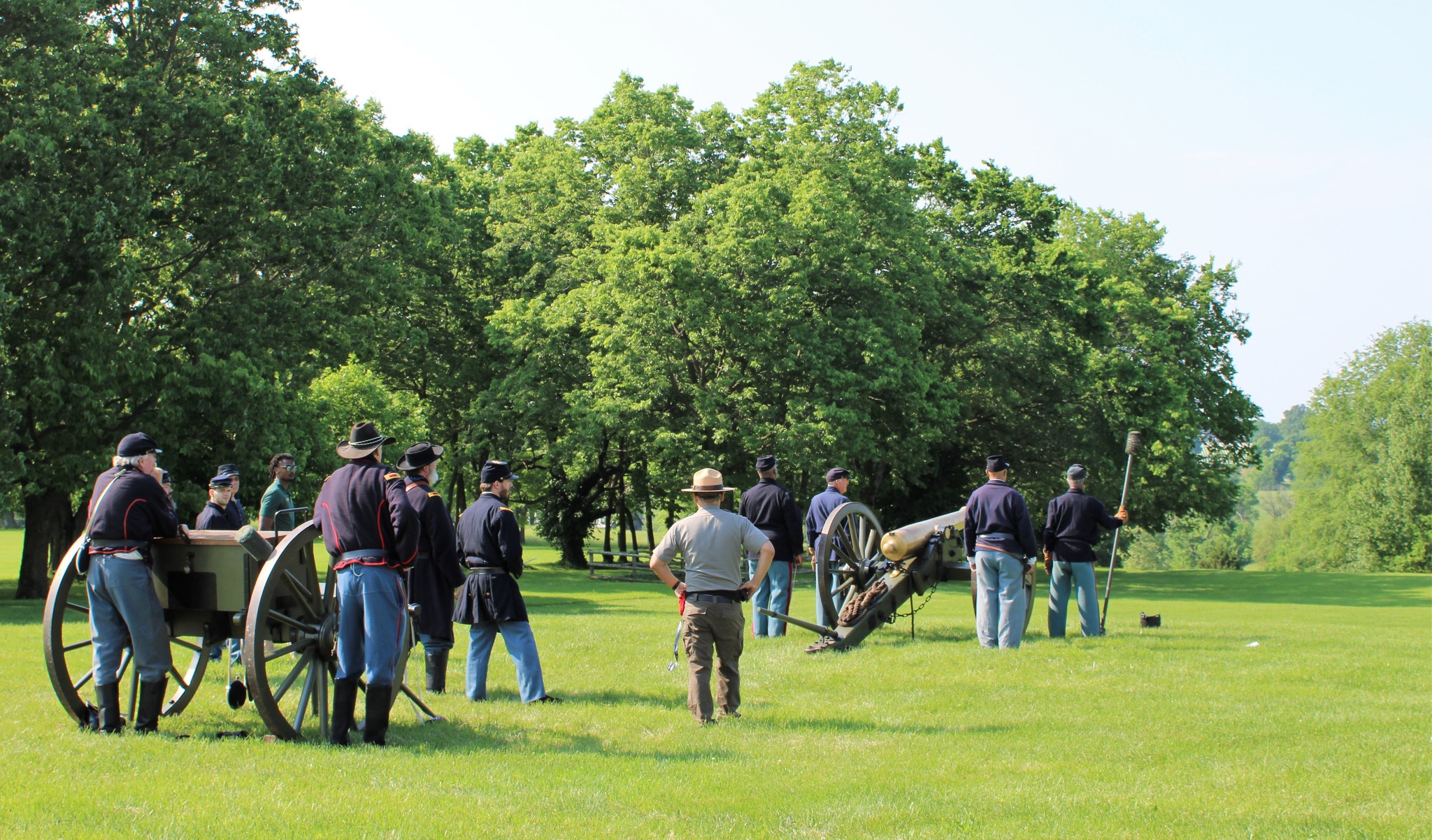This is a detailed landscape photograph capturing a Civil War reenactment set in an outdoor park on a sunny day. Central to the image is a park ranger, identifiable by his gray and khaki uniform, lanyard from his pants, and Smokey Bear-style hat. The ranger stands with his hands on his hips between two groups of reenactors – all dressed in navy blue jackets and light blue pants reflective of Civil War attire.

In the foreground, four soldiers surround a brass cannon. On the right, one soldier, wearing a cowboy-style hat, is holding a cannon ramrod used to load the cannon. Next to him is another reenactor in a dark blue jacket and light blue pants, identifiable by his private's cap. To the left, a white man in a blue shirt stands in front of a black man dressed in a dark blue jacket, light blue pants with a red stripe, and a matching hat.

The background group features more reenactors. Prominently, a man in a dark blue jacket, long light blue pants, and black shoes wears a military cap. Beside him stands a white man with a beard and a minister's cap, dressed in a similar blue outfit. Another character, a black man in civilian clothes and sunglasses, looks directly at the camera. Completing this group is a white man with a private's cap and a blue jacket. In this setup, a storage chest sits between two wheels, hinting at the provisions and gear used during the reenactment.

In the background, tall, lush trees and a clear blue sky without clouds frame the scene, enhancing the historical ambiance of the reenactment. The grassy field in the foreground completes the setting, with light filtering in from the left, casting a natural glow on the participants. All individuals appear to be facing away from the camera, towards the right, possibly waiting for the reenactment to commence or observing something off-frame.